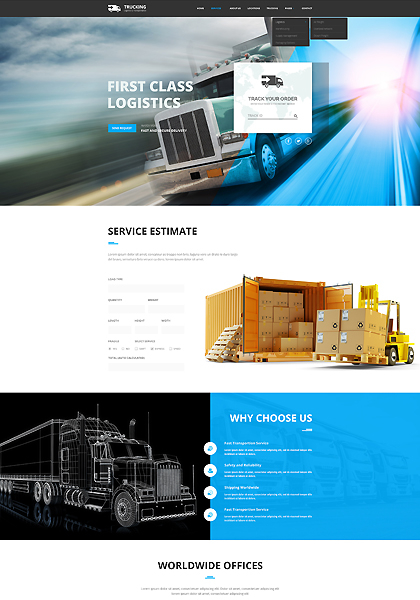Screenshot of a logistics company’s website. At the top, a horizontal black menu bar stretches across the entire width of the image, though the company name is not clearly readable. Below the menu bar, an image of a truck is prominently displayed, facing towards the lower-left corner. Just underneath this image, on the top right, there is a white box labeled "Track Your Orders" which also features a truck icon. To the left of this white box, the text "First Class Logistics" is visible, accompanied by a blue button, with some additional wording nearby.

Beneath the truck image, a white section titled "Service Estimate" occupies the central area, featuring input text boxes presumably for user interaction. To the right of the "Service Estimate" section, an image of a cargo box containing smaller cardboard boxes is displayed. Further down the page, there is a section labeled "Why Choose Us," offering detailed insights about the company's unique selling propositions.